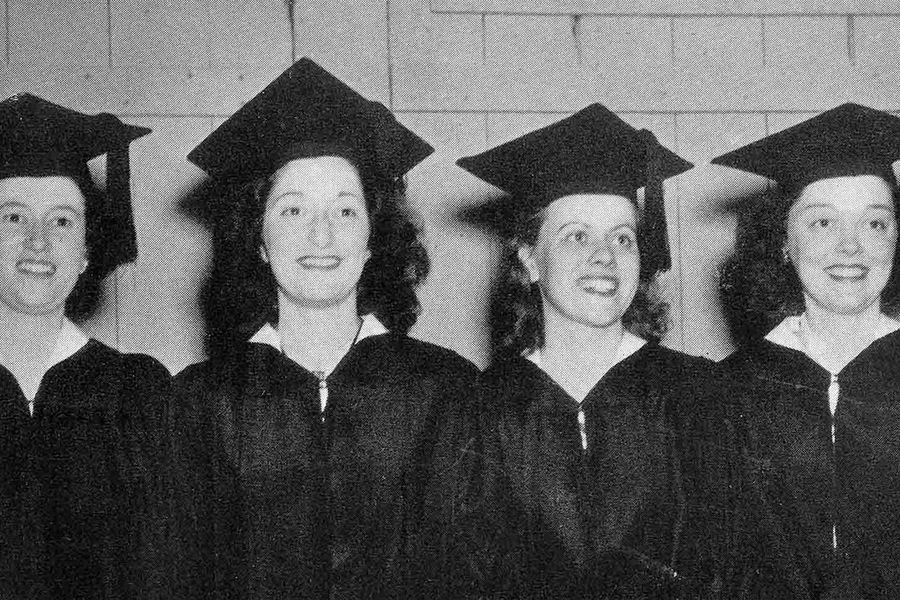This is a grainy, black and white photograph capturing a joyful moment from the past. The image features four young women who have just graduated, standing in a row against a detailed wooden wall, reminiscent of a barn with vertical and horizontal panels. These women are all wearing dark-colored graduation gowns with white collars, and matching square graduation caps with dark tassels that hang over the left side, signifying they have completed their ceremony. Each woman has shoulder-length, dark hair and wears a broad, happy smile, posing proudly for the camera, with their eyes mostly directed slightly off to the right, suggesting multiple photographers. Subtle wear and light scratches are visible on the bottom right side of the photograph, adding to its vintage charm.